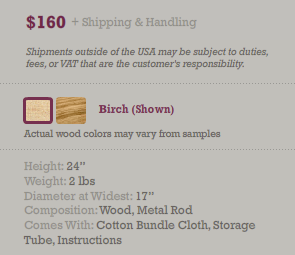Here's a cleaned-up and detailed caption for the described image:

---

The screenshot showcases a product against a light taupe gray background. At the top, "$160" is prominently displayed in a purple-burgundy font. Below this, in a slightly darker shade of the same background color, the text reads "Plus Shipping & Handling", with both "S" and "H" capitalized and "and" represented by an ampersand.

Further down, the caption warns, "Shipments outside of the USA may be subject to duties, fees, or VAT at the customer's responsibility." 

The image illustrates two versions of the product: one in a birch finish and another in a warmer, honey-toned color. The birch option is highlighted with a burgundy-purple outline and labeled "Birch (Shown)" with both "B" and "S" capitalized.

Additional information includes a disclaimer that "actual colors may vary from samples." Specifications such as height, weight, and diameter at the widest point are provided. The product comes with a cotton bundle, cloth storage tube, and instructions.